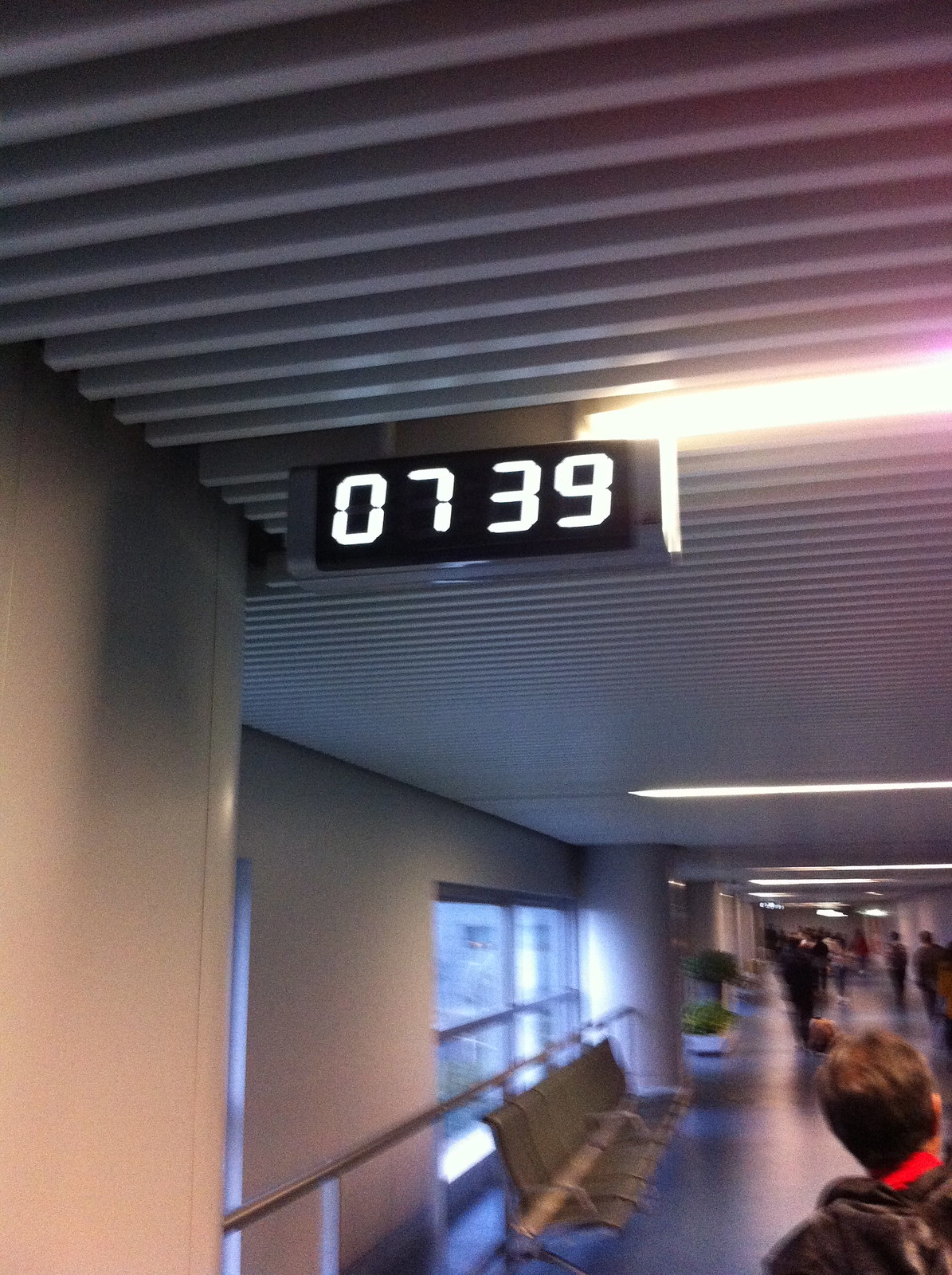The image depicts a bustling airport terminal, characterized by a modern design and a sense of movement. A large clock mounted on the wall prominently displays the time as 7:39, though it does not specify whether it is a.m. or p.m. In the center of the scene, large windows allow natural light to flood in, casting a bright ambiance over the area. Arranged in front of the windows are several rows of seats, providing a resting place for travelers.

In the foreground, a man with a red-collared shirt and a backpack strides through the terminal, capturing a moment of transit. Around him, other passengers are actively engaged in various activities—some are pulling luggage, while others stand in small groups, possibly engaged in conversation or checking their surroundings.

A notable feature in the middle of the hallway is a large plant, adding a touch of greenery to the scene and breaking up the otherwise architecturally-focused space. Overhead, the ceiling is designed with scalloped lines and indentations, accentuated by fluorescent lights that create a dynamic pattern across the expanse. The combination of natural and artificial light, along with the modern ceiling design, contributes to the contemporary and efficient atmosphere of the terminal.